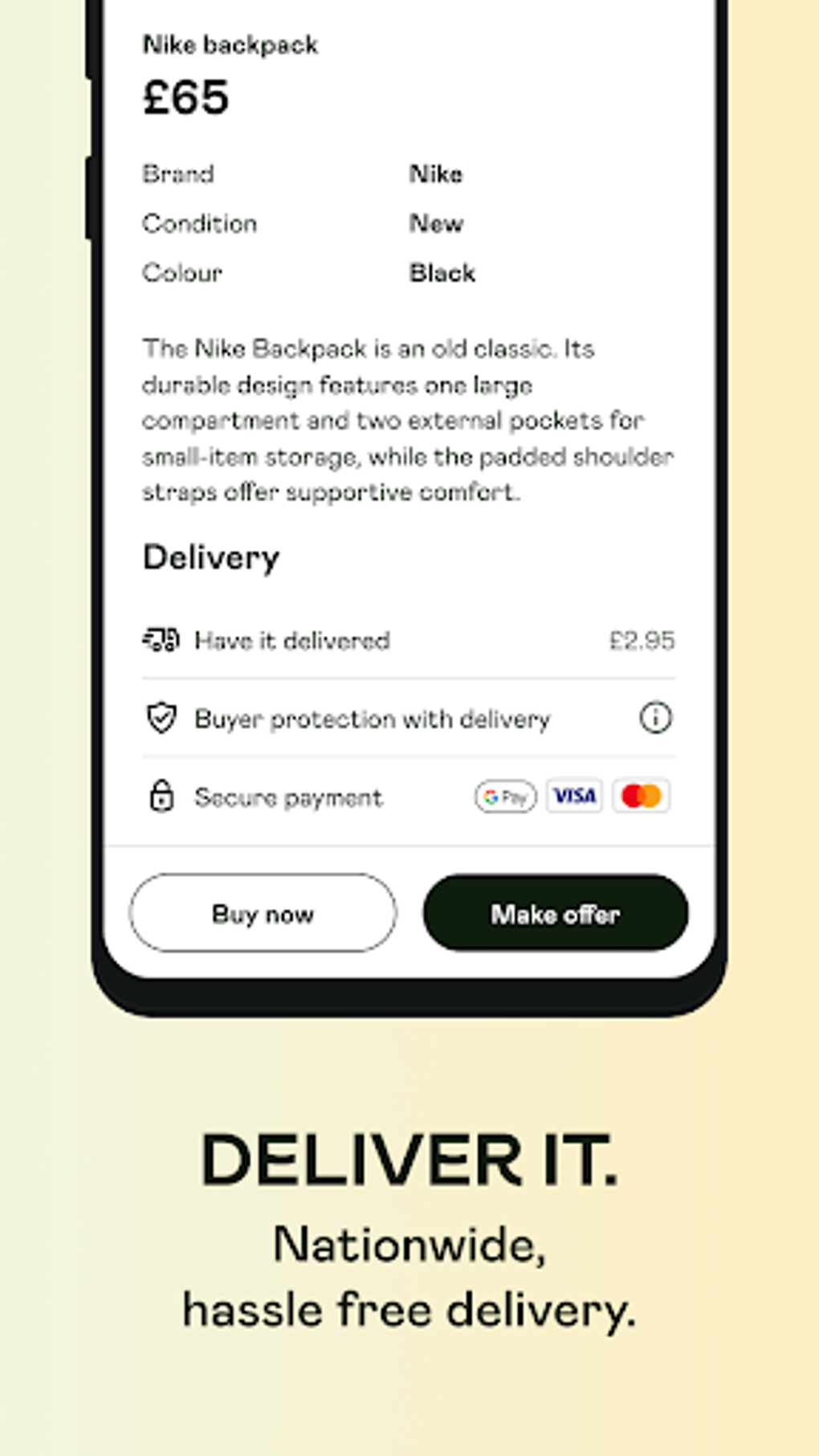This caption provides a vivid description of the image, highlighting the main elements in detail:

---

Screenshot of a mobile app interface displayed on a smartphone, emphasizing that it features a product listing from Nike. The phone, shown in its entirety, has visible volume and power buttons on the left side. The screen displays a Nike backpack priced at £65, set against a white background. The backpack is new and black in color. 

A brief product description notes that this backpack is a classic, durable model featuring two external pockets for small item storage and padded shoulder straps for comfort. The delivery cost is £2.95, which includes buyer protection and secure payment options, with support for GPay, Visa, and MasterCard.

At the bottom of the app screen, there are two interactive buttons: a white "Buy Now" button and a black "Make Offer" button. Beneath the phone, on the poster background, which is peach-colored, there's bold, black text reading "Deliver It", with smaller black text below stating "Nationwide hassle-free delivery".

---

This description thoroughly captures the elements and context of the image, providing a clear and comprehensive visualization for readers.